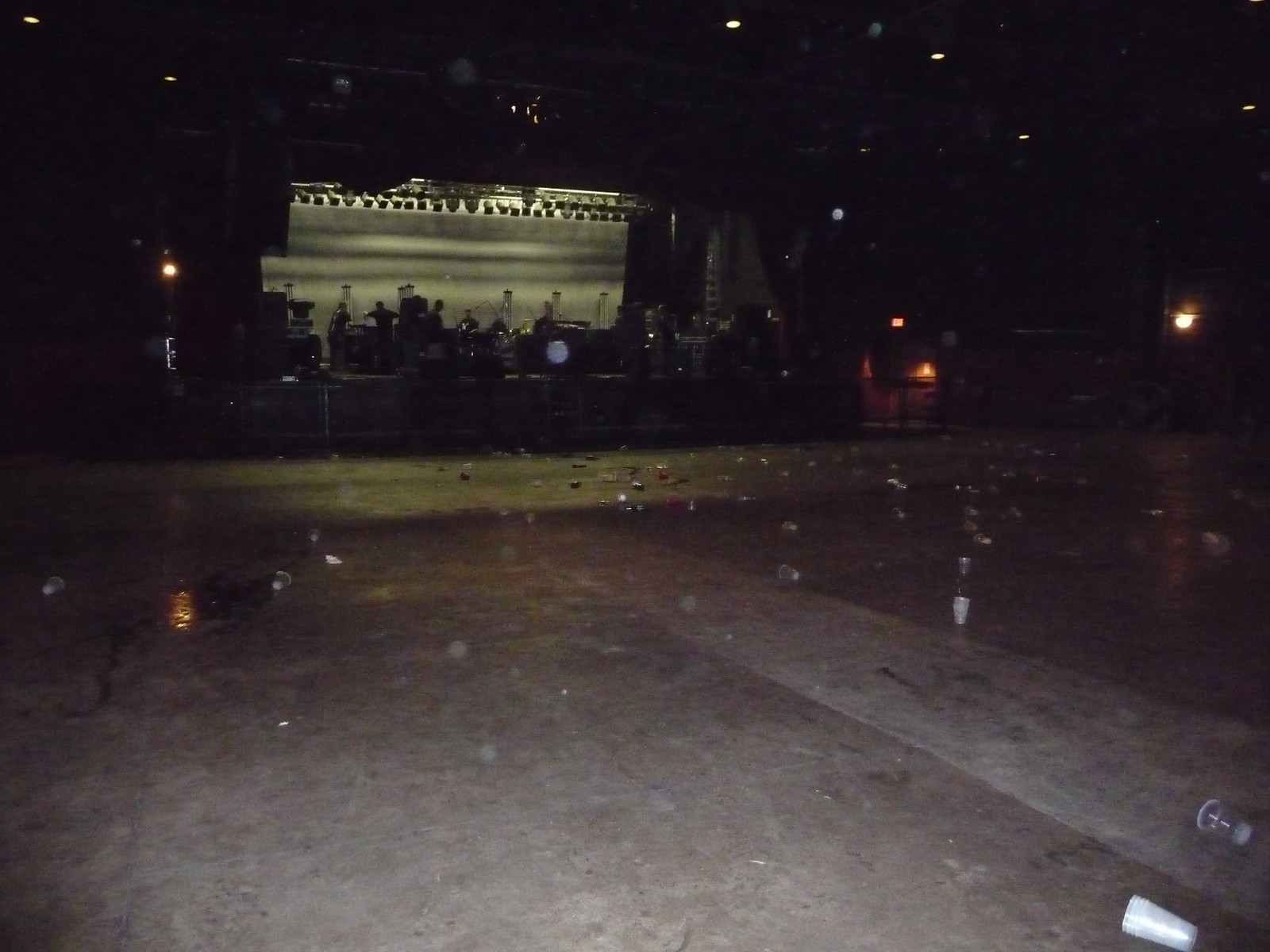An empty ballroom is depicted in the image, bathed in a post-event atmosphere. Musicians linger on the stage, appearing to pack up their instruments. Various musical instruments lie scattered across the stage, under dozens of mounted lights that provide a vivid backdrop. The foreground showcases a barren dance floor, free of chairs but littered with cups and debris. The concrete floor, devoid of any rugs, exhibits a glossy finish that reflects the stage lights. In the background, columns flank the stage, contributing to the room's ornate aesthetic. The combined reflections from the floor and the lighting above create a striking visual contrast in the seemingly deserted space.